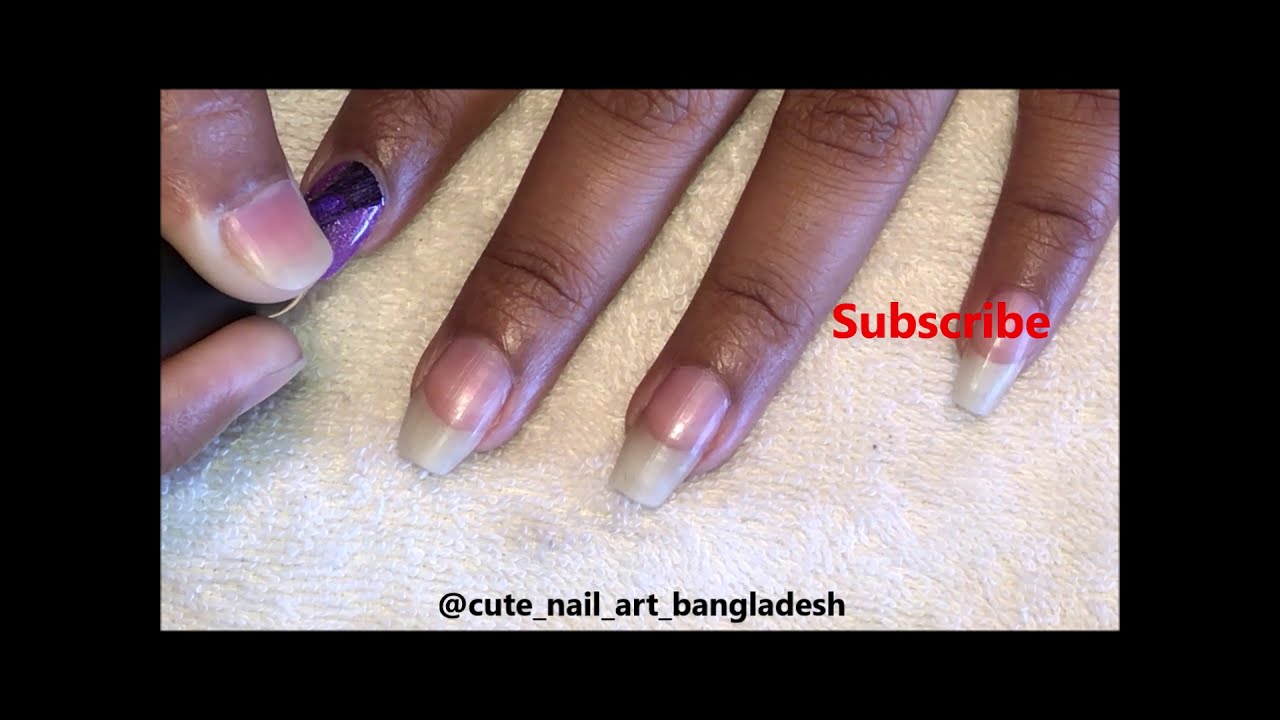In this close-up screenshot of a YouTube video titled "cute_nail_art_Bangladesh," a left hand with dark brown skin and long, bare nails rests on a white towel. The right hand, also with dark brown skin, is meticulously applying a long, purple fake nail to the index finger of the left hand. The scene indicates a detailed nail art tutorial. In bold red letters on the right side of the screenshot, the word "subscribe" is prominently displayed, suggesting a call to action for viewers. At the bottom of the image, the username "cute_nail_art_Bangladesh" appears, indicating the creator's channel or profile name.